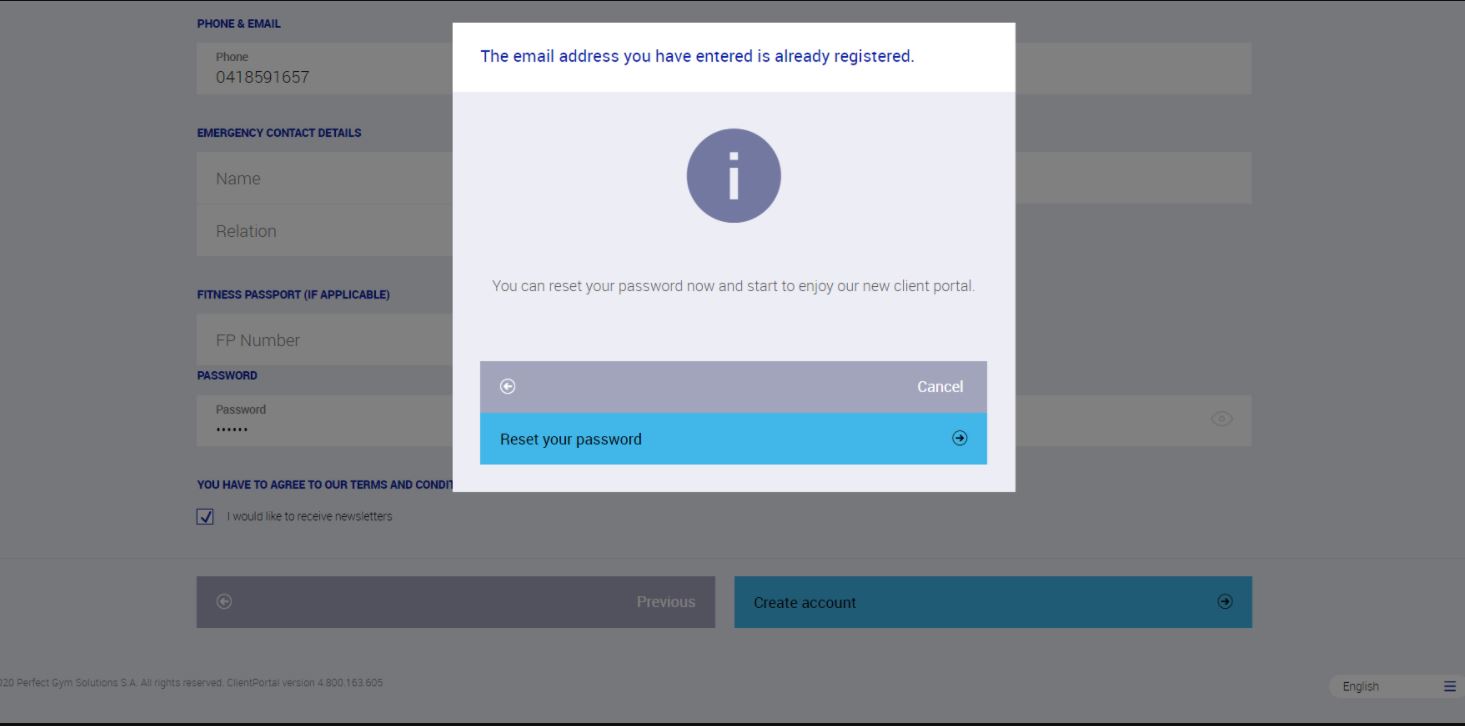This screen capture depicts a registration attempt on a website with a partially obscured background. The background displays several unfilled white input boxes for user details, organized under blue headers. The first header reads "Phone and Email," displaying a sample phone number (041-859-1657) in black text inside the white box. Below, prompts for "Emergency Contact Details," including a name and relation, are present but unfilled.

Further down, another section header in Navy blue indicates areas for entering a "Fitness Passport" number (if applicable), which is not filled in, and a "Password" field showing masked characters represented by asterisks. A gray eye icon next to the password box suggests functionality to reveal or hide the entered password.

At the bottom of the background, the user is prompted to agree to terms and conditions, accompanied by a small white checkbox with a Navy blue checkmark and an option for receiving newsletters. Navigation buttons are displayed at the bottom: a gray "Previous" button with white text and a blue "Create Account" button with black text and an arrow. The language setting shows "English" with a three-line menu icon beside it.

Overlaying this scene, there is a prominent pop-up indicating an issue with the registration. The pop-up, with a Navy blue header, alerts the user that the entered email address is already registered. The message, housed within a gray section, suggests that the user can reset their password and start using the new client portal. Below the message are navigation elements: a gray "Back" arrow with white text labeled "Cancel" and a blue button with black text labeled "Reset Your Password," accompanied by a black forward arrow within a circle.